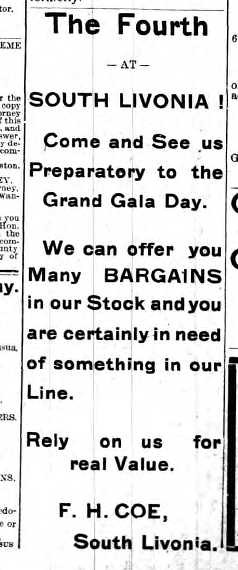The image portrays what seems to be an old newspaper advertisement, possibly classified, with a distinctly vintage appearance that suggests it was photocopied in black and white. The main focus of the advertisement is text-heavy and reads, from top to bottom: "The Fourth at South Livonia. Come and see us preparatory to the Grand Gala Day. We can offer you many bargains in our stock and you are certainly in need of something in our line. Rely on us for real value. F.H. Coe, South Livonia." The text is presented on a plain white background, with certain phrases and names like "South Livonia," "F.H. Coe," and "bargains" emphasized in all caps and larger fonts. The advertisement sits prominently in the center of the image, flanked by snippets of fine print from adjacent newspaper content that are partially cut off and unreadable. The overall dimensions of the image are taller than it is wide, adding to its rudimentary and straightforward aesthetic.